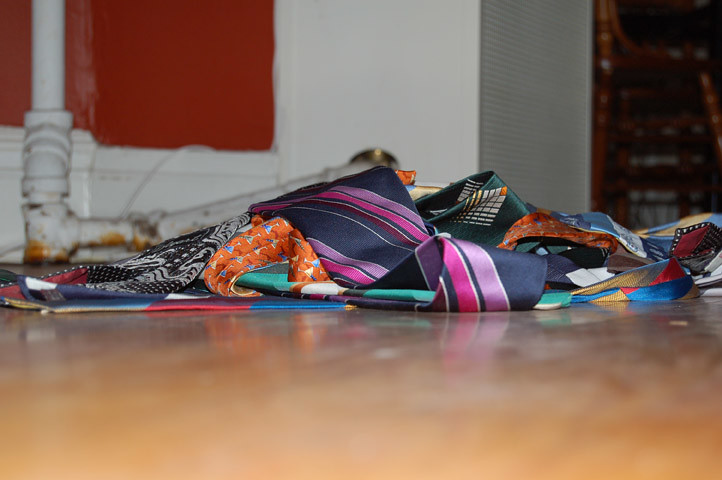This indoor color photograph captures a close-up view of approximately 13 to 14 neckties jumbled in a pile on a neutral brown wooden floor. The ties, appearing brand-new and predominantly silk, feature a variety of vibrant designs: diagonal stripes of black, silver, and magenta; lively orange floral patterns; and intricate green and black decorative scrollwork. Other ties display a color range from aqua blues to blacks with gold trim. This vivid assortment lies in the center of the image, forming a mound with some ties lying flat and most entangled. The foreground of the floor is slightly out of focus, bringing attention to the ties. In the slightly more focused background, a white water pipe climbs up a wall with white trim and an orange center, leading to a radiator heater inside an enclosure. Additional background details include a mix of light beige and red surfaces, with a glimpse of a blackened upper right corner and an opening that might be a closet to the right. The overall scene is an artistic yet chaotic snapshot of patterned and decorative neckties against an everyday setting.